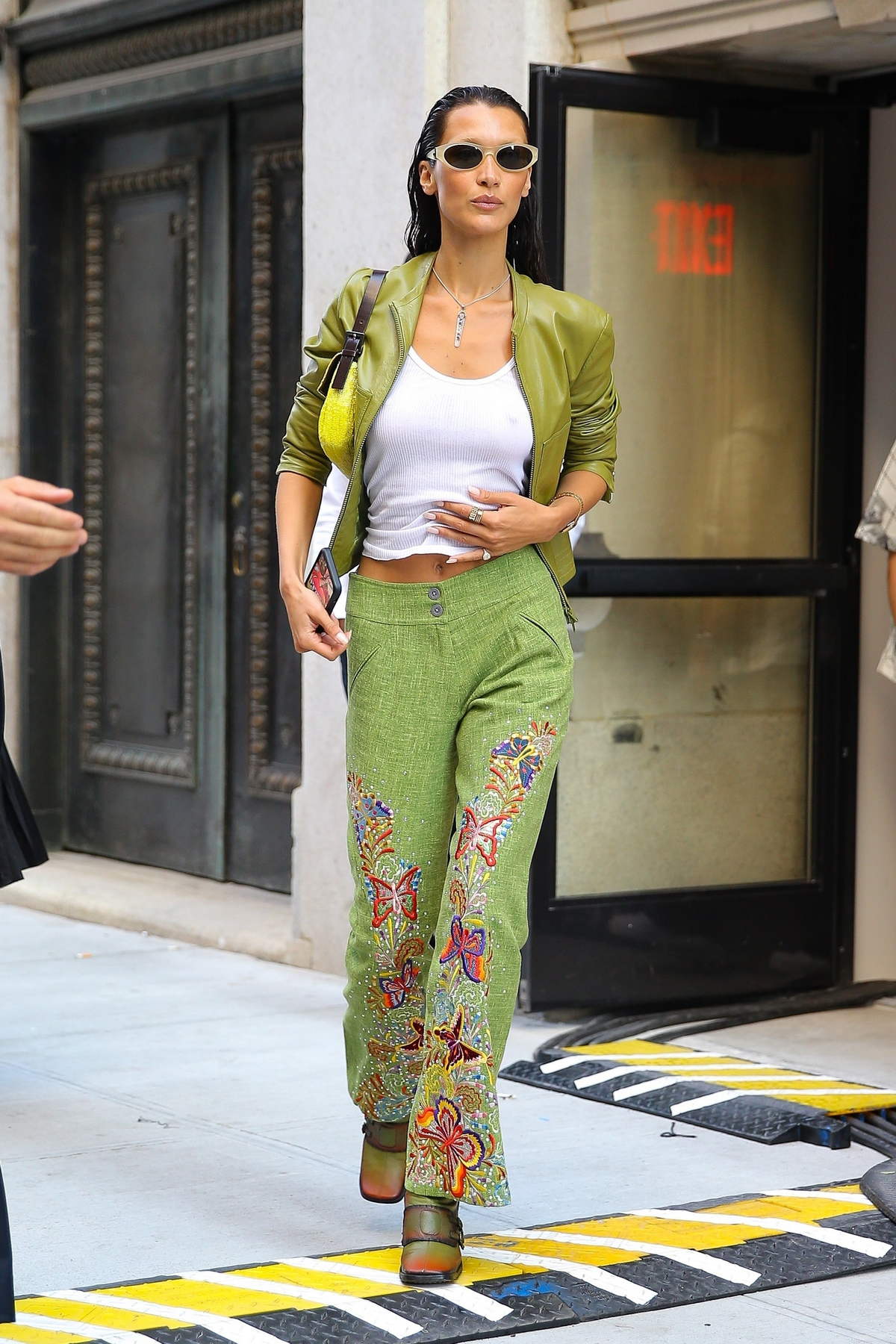This image features a light brown-skinned woman walking outdoors on a sidewalk, facing the camera with her entire body visible. She has long, dark hair styled in slick braids falling behind her shoulders and wears wide oval-shaped dark sunglasses. The woman is dressed in a white low-cut crop top, partially exposing her chest and belly button, under a bright green leather jacket with pushed-up sleeves. She accessorizes with a small silver necklace and a chartreuse purse with brown straps draped over her right shoulder. Her pants are light green and adorned with embroidered butterflies rising from the hem to her thighs. She completes her outfit with green and red shoes. In her right hand, she holds a smartphone. She appears to be stepping out of a glass door with a red "EXIT" sign reflected on it and walks over a textured mat covering cables on the ground. Notably, the shadows around her feet seem incorrect, suggesting the image might be AI-generated.